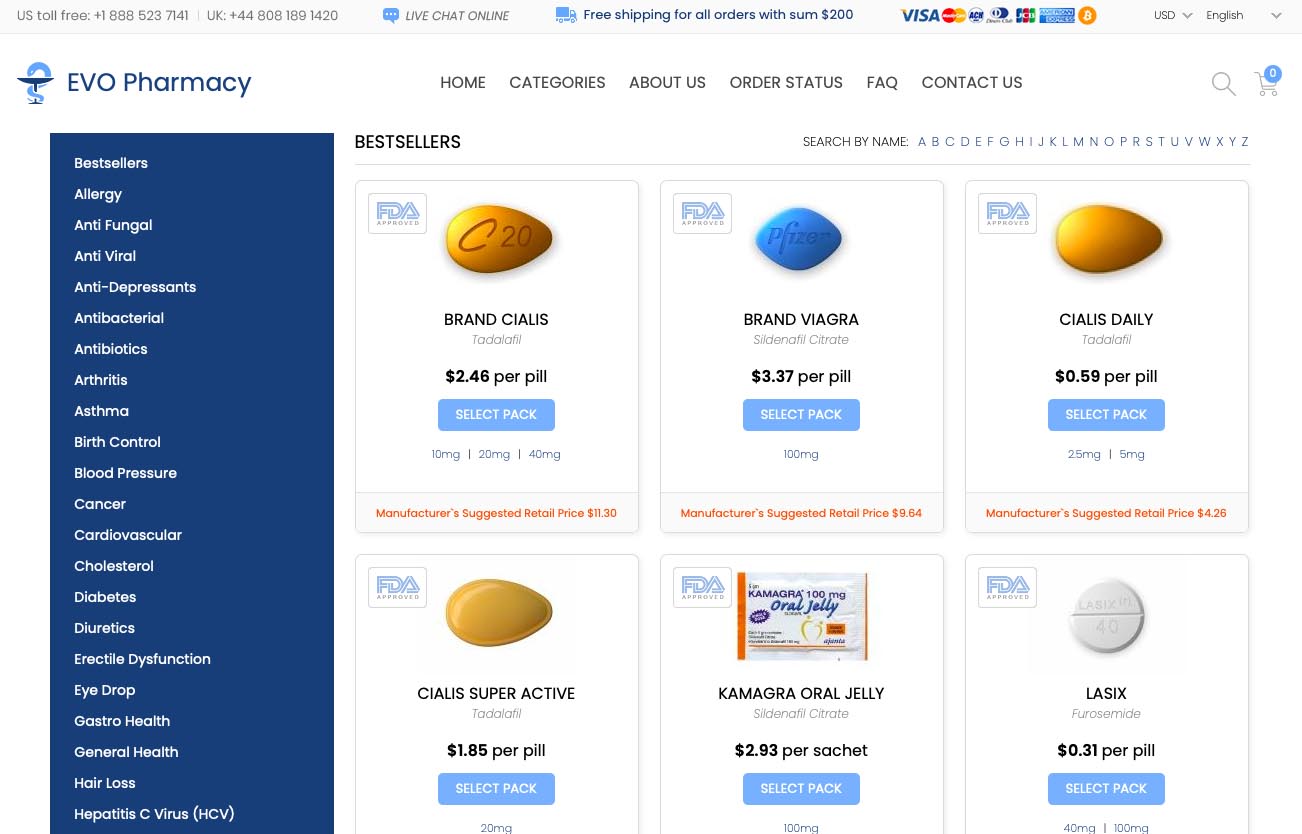This screenshot from the EVO Pharmacy website features a rectangular layout, predominantly showcasing the pharmacy's offerings and best-selling products. On the left side of the image, "EVO Pharmacy" is prominently displayed in dark blue text, alongside a turquoise icon. Below this header, there is a tall, rectangular sidebar listing various pharmaceutical categories. These categories, written in white text, include allergies, antifungal, antivirus, antidepressants, antibacterial, antibiotics, cancer, cardiovascular, cholesterol, diabetes, diuretics, erectile dysfunction, eye drops, hair loss, and hepatitis C.

In the main section, spanning from the center to the right side of the image, is a list of the pharmacy’s best-selling pills. The header "Best Sellers" is written in black text. The pills are depicted in different shapes and colors: the top row features pills in shades of orange and blue, while the bottom row includes dark yellow and white circular pills. Additionally, there is an image of a pill box among the products. Text throughout the image varies in shades, including whites, dark blues, black, light grays, and occasional orange accents.